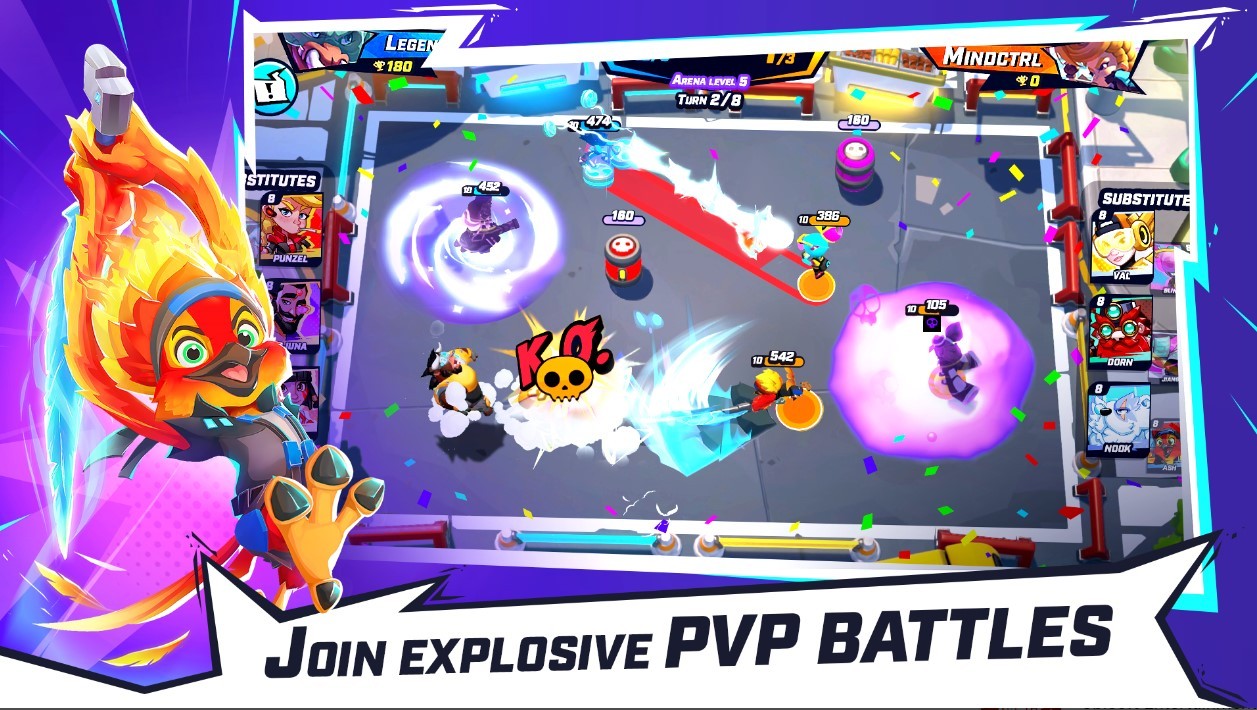The image is a vibrant, cartoonish-style illustration reminiscent of a video game. Dominated by bold colors like purple, red, orange, and blue, it features a battle game scenario inviting viewers to "Join Explosive PvP Battles." On the left side stands an animated parrot-like bird with red flame-like hair and an orange face, gripping a sword shaped like a long feather over its back. The middle of the scene resembles a battleground akin to a Pokémon arena, complete with pinball-type bumpers and action-indicating clouds. Surrounding this field are square icons showing the heads of different comic-style characters, likely representing waiting or substitute players. The player icons listed on the right and left sides suggest the involvement of six players, with notable names like Mind Control and Legend. Completing the dynamic scene is a vivid bluish-purple background that solidifies the energetic, game-focused atmosphere of the image, which appears suitable for an advertisement or brochure promoting an engaging PvP video game.